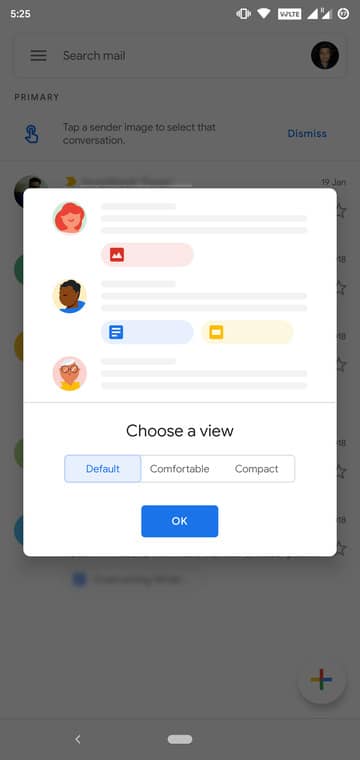This is a screenshot taken on an Android cell phone, showcasing an interface from the Google Gmail application, faintly visible in the background with a dim dark gray hue. At the forefront of the image is a white square pop-up window displaying a "Choose a View" prompt. The pop-up contains three clipart-style icons representing a woman, a man, and an older person, each corresponding to different layout options. Below these icons are three descriptive buttons: "Default," "Comfortable," and "Compact," allowing the user to select their preferred email view. Centered at the bottom of the pop-up is a prominently displayed, blue "OK" button for confirming the selection.